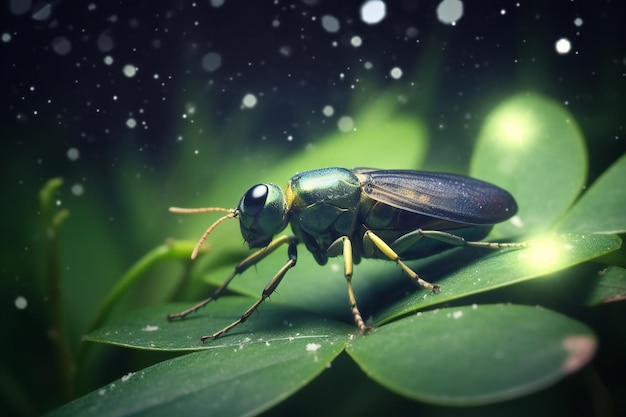This is an extreme close-up image, possibly computer-generated or AI-created, of a green insect that bears some resemblance to a grasshopper but with distinguishing features that set it apart. The insect is perched on a leaf, which seems to be part of a five-leaf clover. The creature has a unique body structure with a notably short abdomen and a pair of intermediate legs in place of the traditional jumping hind legs characteristic of grasshoppers. Its wings, which are black with yellow highlights towards the center, are folded neatly over its back. The insect's upper torso sports a hard, shiny green shell, and its head is green with strikingly large black eyes. Yellow antennae protrude from its head. The background is entirely black with some white specks, possibly resembling dust, giving the whole image an almost surreal, isolated appearance. Only five legs are distinctly visible, though it seems there should be six, hinting at possible image inconsistency.